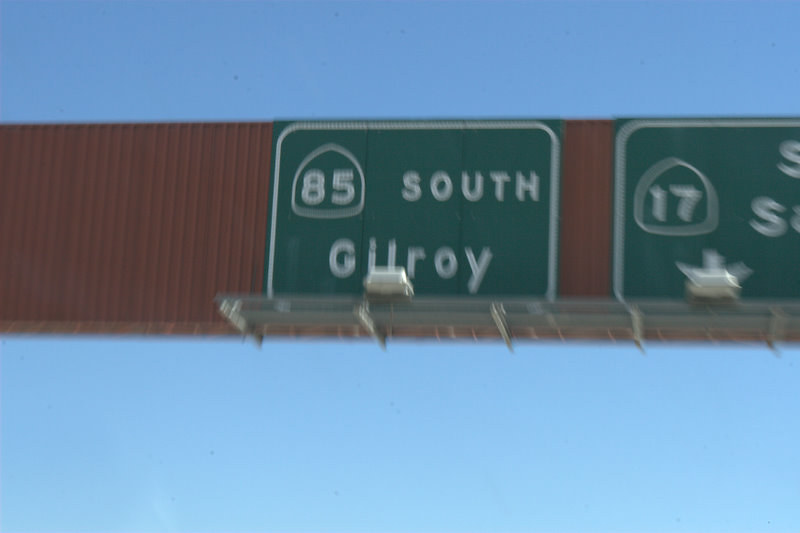The image captures a view looking upward, likely from the perspective of someone in a vehicle passing underneath a signage system on a freeway. The backdrop is a light blue, clear sky. Dominating the frame is a structure that spans the entire width of the photo, appearing reddish-brown and resembling either wood or metal paneling. Mounted on this structure are two green highway signs with white lettering. The larger, square-shaped sign prominently displays "85 South Gilroy" with the number 85 encased in a white circle. Nearby, another green sign shows the number 17 within a white circle, with partially-visible text starting with the letter 'S'. Attached beneath these signs, there is a silver frame extending about six inches, likely housing lamps intended to illuminate the signs at night. The overall setting indicates a freeway environment with clear visibility offered by the bright, daytime sky.